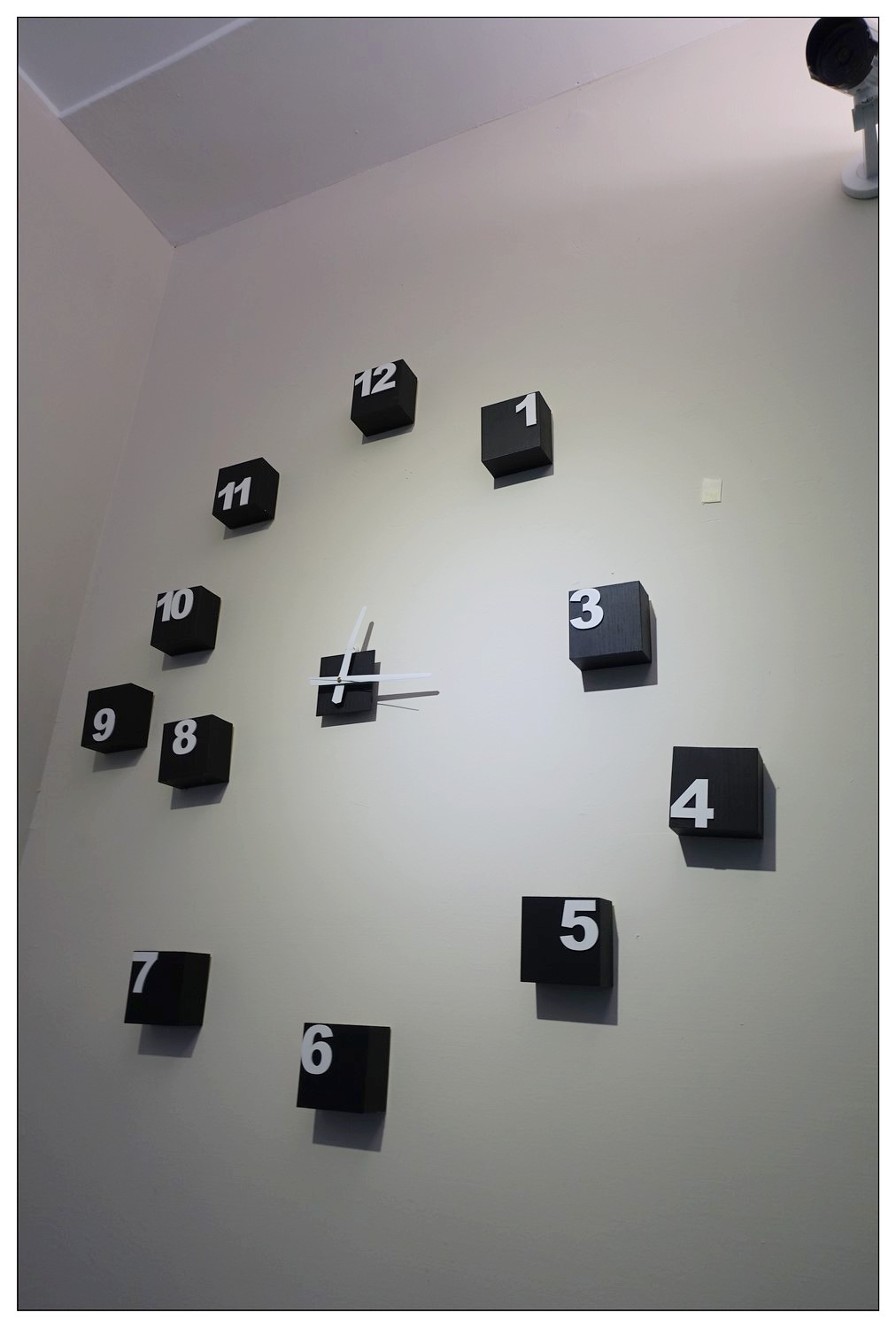This image showcases a unique and modern art-inspired clock mounted on a stark white wall. The clock is composed of 13 black square blocks arranged almost in a circular pattern. Each block represents the hours from 1 to 12 with one additional block at the center, which houses the clock's hands. Interestingly, the number 4 block is protruding slightly to the left, and the number 8 block is positioned more toward the inner part of the circle, creating an asymmetrical yet captivating design. The center block displays the white clock hands indicating the current time, which is 1:15.